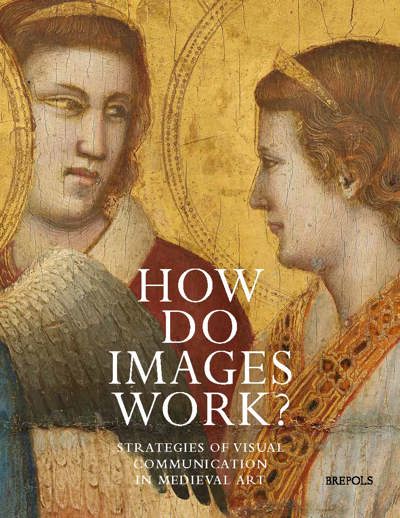The image appears to be a scan of a book cover, featuring a distinctly rectangular poster design. Dominating the background is a detailed section of a medieval painting, characterized by a rich gold backdrop. This painting vividly displays two human figures, adorned in robes, engaged in a meaningful gaze at one another. One figure on the right wears a gold headband over brown hair, adding to the ancient, almost ecclesiastical aura suggested by the art style. Prominently displayed across the top in capitalized, bold white letters is the main title, "HOW DO IMAGES WORK?", with a smaller subtitle beneath it reading, "Strategies of Visual Communication in Medieval Art." The publisher's name, "Brepols," is neatly printed in black in the lower right corner. The cover's color scheme effectively employs strong gold, white, and pink tones to create an aesthetically compelling and historically evocative visual.